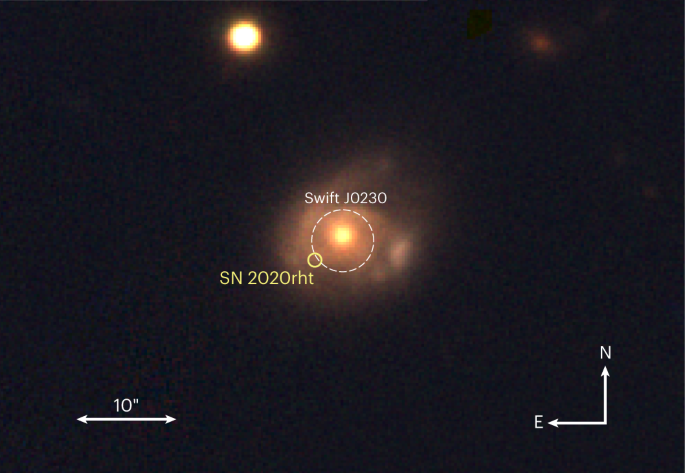The image depicts a vast expanse of space marked by a pitch-black background. In the upper left corner, a glowing orb radiates an orange, yellowish, and whitish light, resembling a sun or star. Moving to the right of this orb, there is a small, scattered reddish-brown area, possibly indicating another celestial object or nebulous region. Below and centered in the image is another glowing orb of a similar orangish hue, surrounded by a circular, cloud-like formation in a slightly different orange and yellow gradient. Encircling this central orb is a dotted line, highlighting it with annotations that read "Swift J0230" above, and "SN2020RHT" below. In the bottom left corner, there is an arrow labeled "10 inches," while the bottom right corner features a partial compass with markings pointing to the "N" for north and "E" for east. This detailed depiction suggests a celestial scene viewed through a telescope, capturing nuanced details of objects in space.